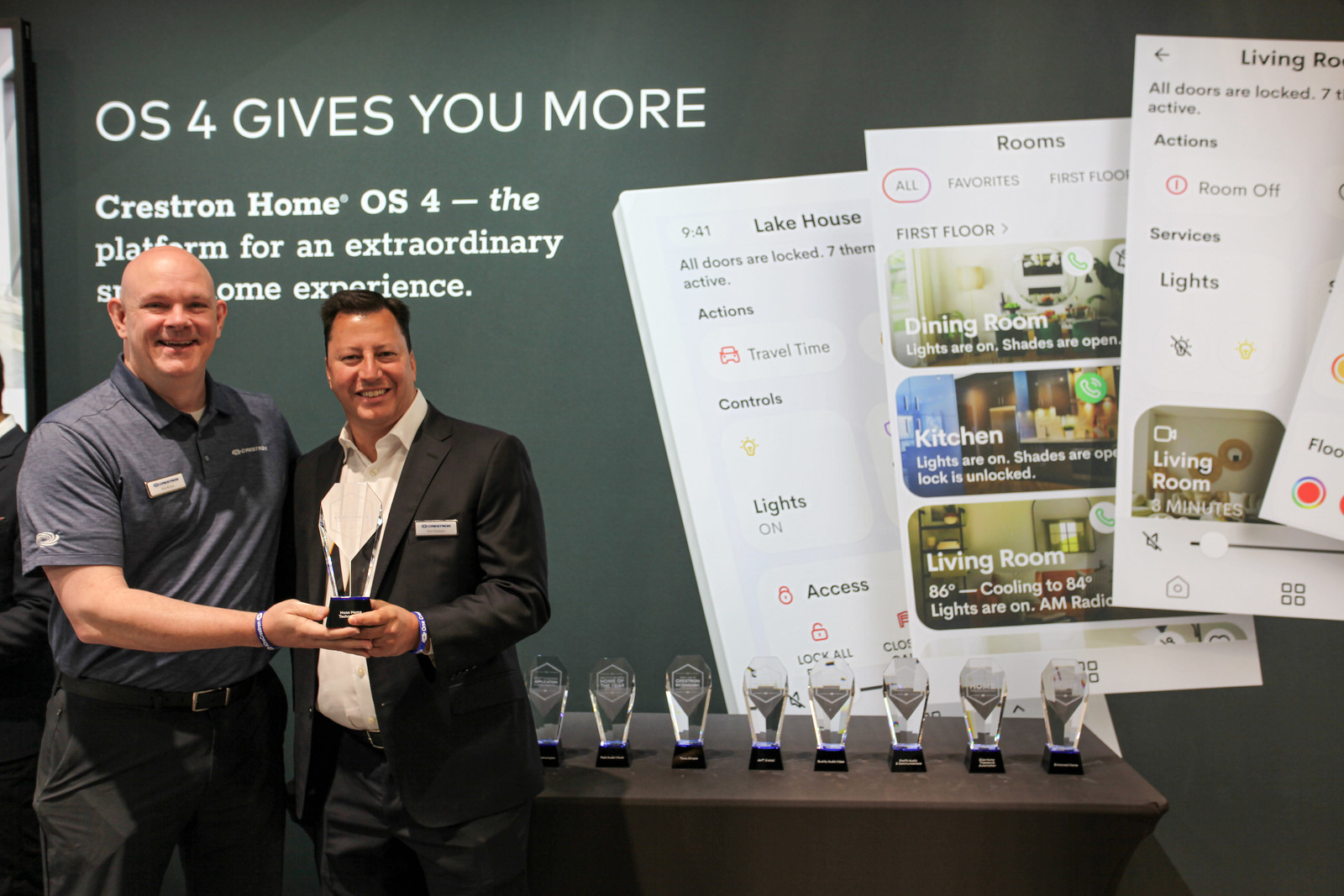In the photograph, two men stand side by side on the left-hand side of the frame, holding a phone together. The man on the right is dressed in a black suit with a white collared shirt and black pants, and has black hair. The man on the left, who is bald, wears a blue polo shirt paired with black khakis and a name tag. Behind them, a white projection screen displays the text "OS4 gives you more, Crestron Home OS4 the platform for an extraordinary" with the rest of the sentence obscured by the men. The screen also shows various screenshots of an app interface, labeled with terms such as "Rooms," "Living Room," "Lake House," "Actions," "Controls," and "Lights." In the background, a gray table holds multiple clear awards. The overall scene suggests a presentation or award ceremony for a home automation platform that offers advanced control over home lighting and security systems.